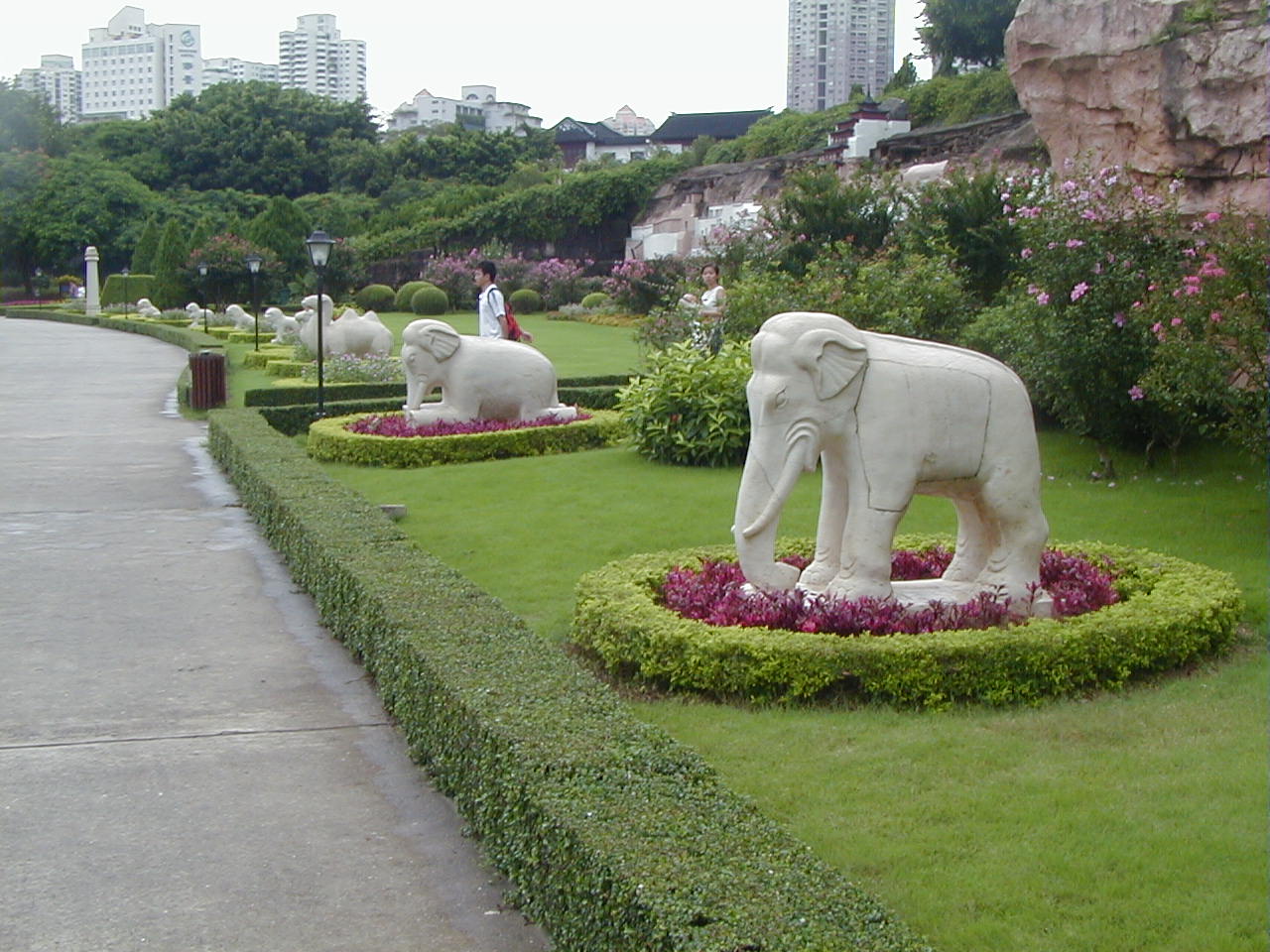The photograph captures a serene urban park set against the backdrop of a bustling cityscape with tall white high-rise buildings, possibly apartments or offices, that soar into an almost white sky. The park features lush greenery with trees, well-manicured lawns, and low, neatly trimmed hedges. Among these natural elements, there are various concrete statues of Thai-style white stone elephants, some standing while others are kneeling in genuflection. These statues are strategically placed in circles of short green hedges interspersed with vibrant red and violet flowers.

Curated gardens with blooming bushes of pinkish flowers and a wall of brownish rock add to the visual appeal. Pathways paved with segmented concrete slabs meander through the park, flanked by lantern-style electric lights on black poles. Two East Asian individuals, a boy and a girl dressed in white shirts—the man carrying a reddish pouch—are seen walking along the path. Additional animals, including white stone camels and lions, are visible in the distance. Further adding to the park's charm is a brown garbage can centrally located, ensuring cleanliness in this picturesque setting.